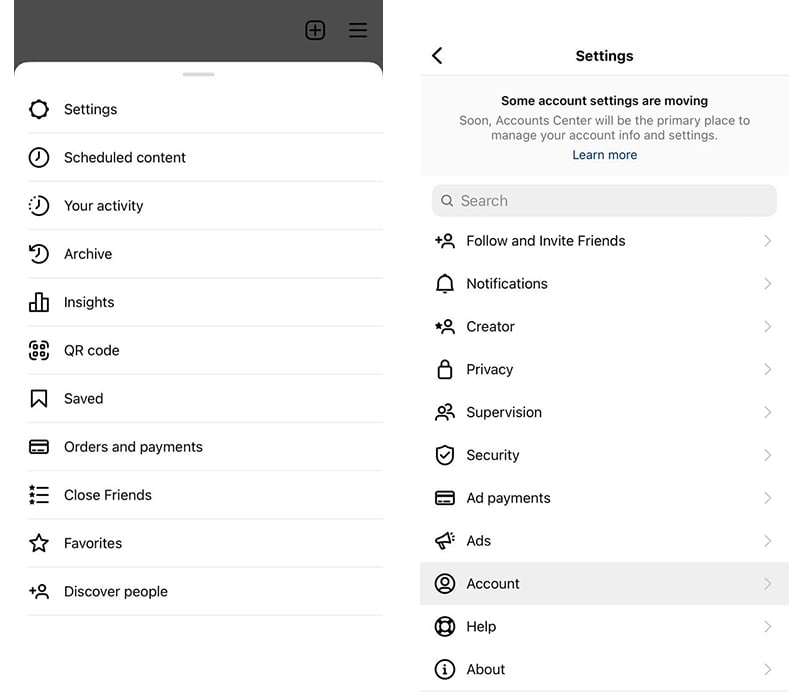The image depicts a smartphone screen showcasing various settings and options within an application. At the top is a gray rectangular button labeled "Settings." Below it, there is a section with a line that reads "Schedule Content Clock" and another option "Your Activity." The screen also features a rotating icon that directs you to "Archive Insights," represented by a bar graph illustration, followed by the "QR Code" option.

A prominent banner displays "Saved," and a card beneath it is labeled "Orders and Payments." Other options listed include "Close Friends," "Holiday Star," "Favorites," and "Discover People." In the top left corner, the Settings section is reiterated, with a note saying "Texas" and mentioning that some account names are currently active. There's an announcement that "Soon an account center will be the primary place to manage your account," along with a clickable "Settings" link to "Learn More."

Additionally, a gray oval search bar is displayed, accompanied by a plus icon and a prompt "Follow and Invite Friends." The screen provides further settings including "Notifications," "Creator," "Privacy," "Supervision," "Security," and "Payments." A final gray rectangle includes an "Account" option. Toward the end, there's a lifesaver icon indicating "Help," and a circle with an "i" in the center for "About."

This detailed look confirms that the image is indeed of a smartphone screen showing various settings and features of an app interface.